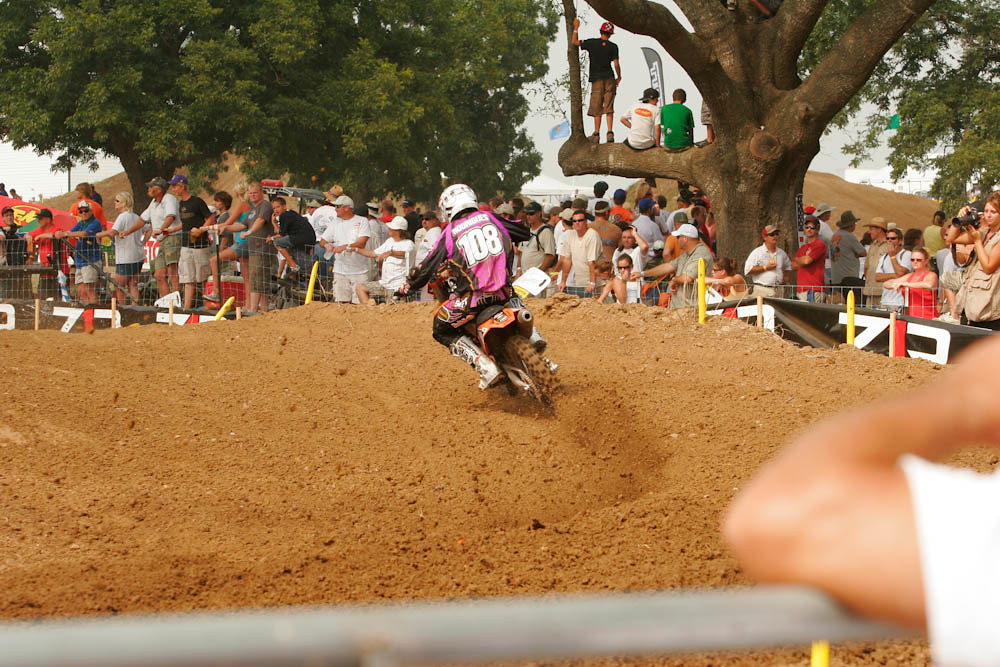In this vibrant outdoor photograph of a motocross race, an orange motorcycle, driven by a rider in a white helmet and distinctive pink long-sleeve shirt with the number 108 in white, takes center stage. The rider, also clad in black pants and thick white boots, is seen maneuvering a dirt track, leaning into a bend as they head slightly left. The backdrop reveals a bustling crowd of spectators lined up behind a fence, eagerly following the race. A metal railing with an out-of-focus arm propped on it occupies the lower right foreground. Dominating the scene are two imposing trees: to the left, a tree with dark green, dense leaves and a broad crown, and to the right, a massive tree with thick branches, one of which supports three or four boys climbing and sitting, providing them with a unique vantage point. The sky overhead is overcast, casting a diffused light over the lively scene.